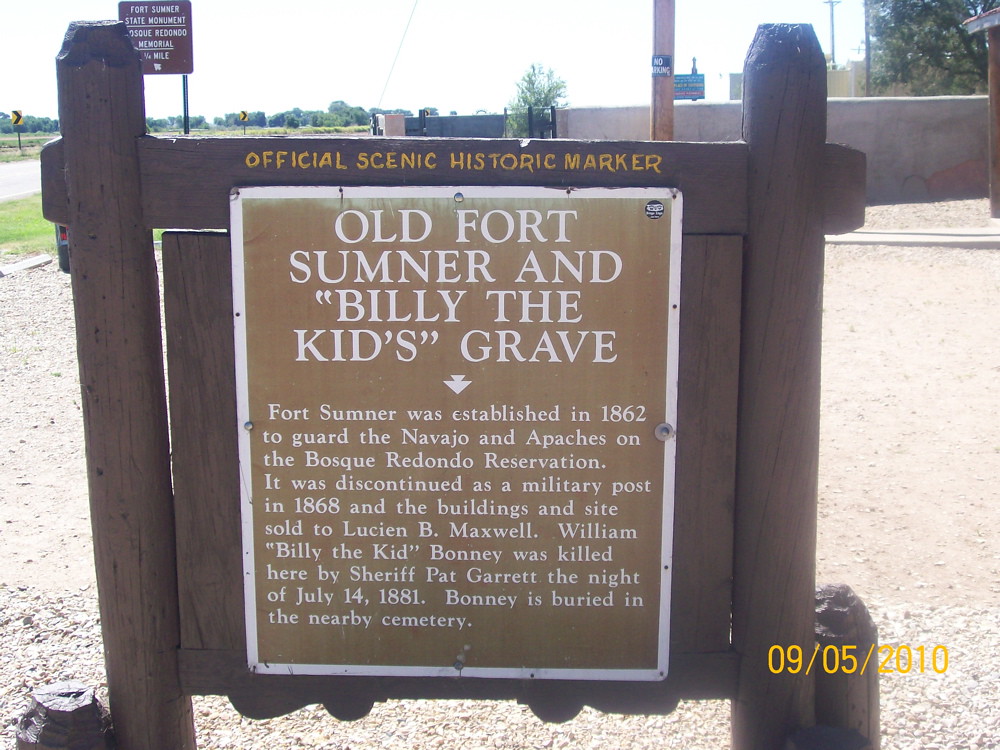The photograph, taken on September 5th, 2010, captures an official scenic historic marker set against a somewhat washed-out daytime sky. Central to the image is a weathered, brown wooden signpost to which a metal plaque is bolted. The wooden post displays a handwritten yellow inscription that reads "Official Scenic Historic Marker." The plaque itself is light brown with a white border and features white lettering that announces "Old Fort Sumner and Billy the Kid's Grave." The detailed inscription on the plaque narrates the history: "Fort Sumner was established in 1862 to guard the Navajo and Apaches on the Bosque Redondo Reservation. It was discontinued as a military post in 1868, and the buildings and site were sold to Lucian B. Maxwell. William 'Billy the Kid' Bonney was killed here by Sheriff Pat Garrett the night of July 14th, 1881. Bonney is buried in the nearby cemetery." In the background, a road can be seen to the left, while a low, brownish brick wall and a black metal gate extend to the right. The foreground is primarily covered in gravel and sand, emphasizing the historic and rustic atmosphere of the location.